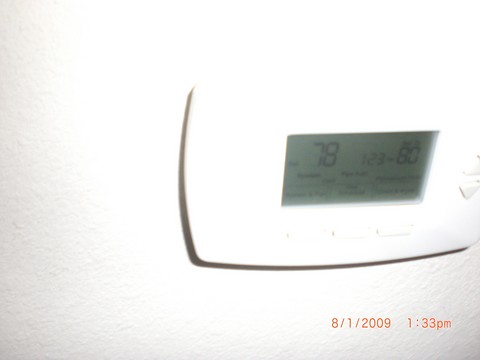The image features a slightly out-of-focus thermostat, illuminated by a very bright light, resulting in a noticeable dark shadow on the left and bottom sides of the device. The thermostat has a large plastic panel, which includes a central display screen showing the number "78" and partially readable text resembling "123-80." Due to the brightness and blurriness, additional text on the display is indiscernible. Positioned to the right of the display are two triangular buttons—one pointing upwards and the other downwards—typically used to adjust the temperature settings. Below the display, there appear to be three or possibly two indistinct buttons, faintly visible due to the shadow. At the bottom of the image, a time stamp is clearly marked in red, reading "8-1-2009 1:33 PM," indicating either August 1st, 2009, or January 8th, 2009, at 1:33 PM.